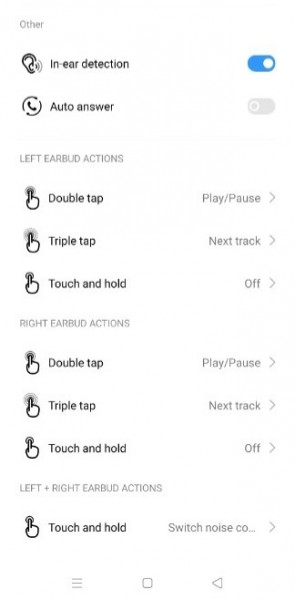This screenshot displays the settings menu for a pair of wireless earbuds, specifically focusing on customizable actions. The "In-Ear Detection" option is highlighted in blue with a checkmark, indicating that this feature is enabled. Other options, such as "Auto Answer" and "Double Tap" and "Triple Tap" gestures, remain unchecked. The interface allows users to personalize their listening experience by choosing which features to activate, ensuring optimal functionality tailored to user preferences.